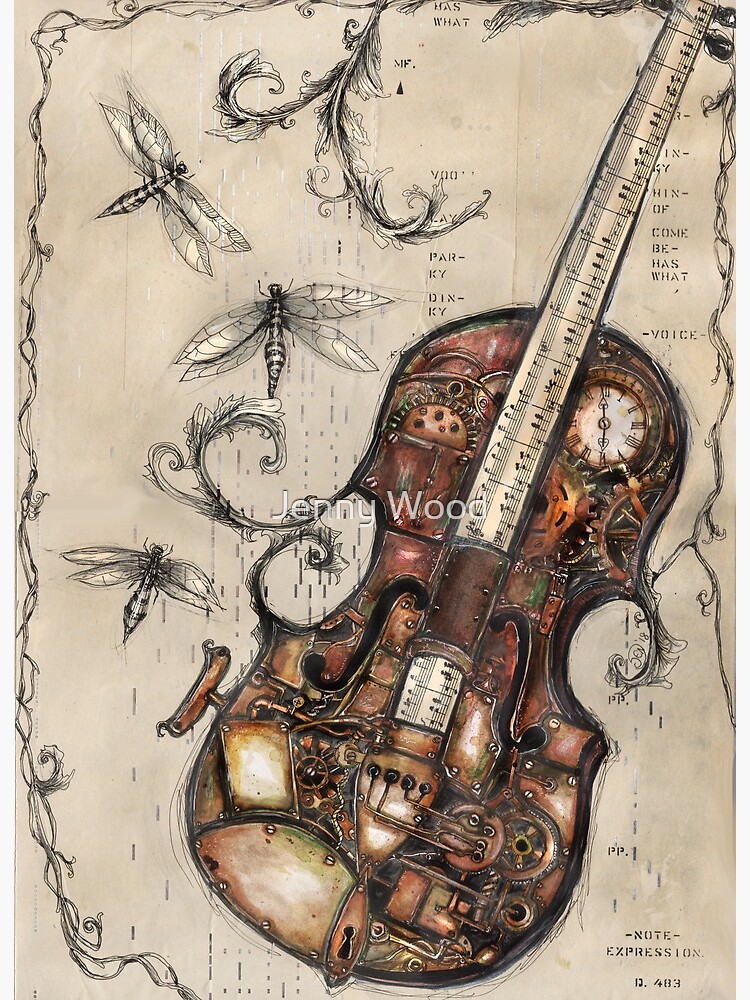This poster-sized artwork depicts a brass-colored, mechanical-looking violin against a creamy tan background. The violin is intricately designed with visible gears, keyholes, and various metal parts, giving it an almost steampunk aesthetic. The neck of the violin is adorned with white musical notes, resembling a tape measure that adds an artistic touch to the instrument. Clocks and Roman numerals are strategically placed on the violin, contributing to its complex design. 

Surrounding the violin, black and white fireflies can be seen buzzing around the upper left side of the poster, alongside curly cues and intricate vines that both wrap around the border and descend from the center. Small black typed fonts with words can be found on both sides of the neck of the violin, adding another layer of detail to the composition. 

In the bottom right corner of the poster, the logo reads "Knight Expression," followed by "D4B3." The combination of these elements creates an evocative and fascinating image, blending musical instrument design with surreal, mechanical elements and natural motifs.